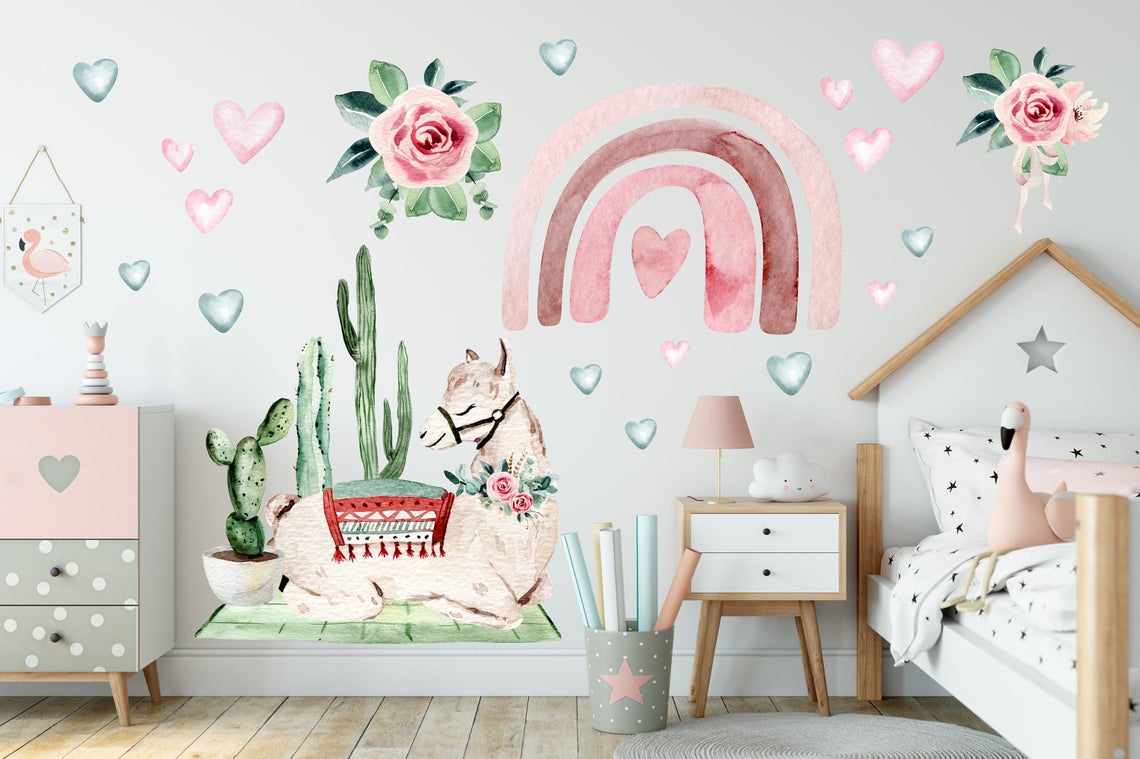The photograph depicts a charming children's bedroom featuring light-colored wooden plank flooring. The walls are adorned with playful decals including pink and green hearts, pink roses, and a vibrant pink rainbow. Central to the decor is an endearing illustration of a lounging llama with a floral collar, surrounded by green cacti. 

On the right side of the image is a cozy white bed with a distinct house-shaped headboard, complete with a brown roof and a cut-out star in the middle. The bed is dressed in white sheets patterned with black stars, and a cheerful stuffed flamingo sits atop it. Next to the bed is a light wooden nightstand with two white drawers. It holds a cloud-shaped lamp and a pink lamp with a gold base.

Adjacent to the nightstand is a gray wastebasket decorated with white dots and a prominent pink star, filled with various rolled-up papers. On the left side of the room stands a coordinating gray dresser with white polka dots, featuring a pink drawer with a gray heart cutout. A circular gray rug lies just to the left of the bed, adding a cozy touch to the space. The thoughtful arrangement and whimsical decorations make the room look almost like an advertisement for a children's bedroom renovation company.